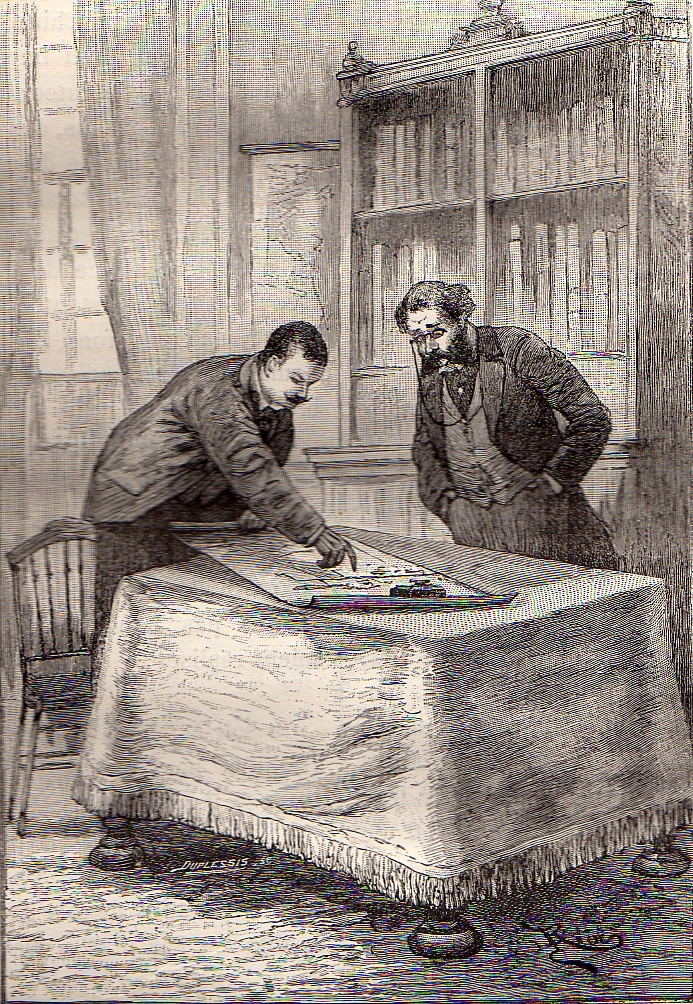This detailed black and white drawing, created with fine etch marks and cross-hatching, captures a moment inside a Victorian or pre-Victorian home. The taller-than-wide rectangular image reveals two men intensely examining a large document, possibly blueprints or instructional plans, spread across a square table in the foreground. The table is dressed in a fringed tablecloth that descends almost to the floor, revealing three circular feet at the bottom. 

To the left, a man with short black hair, a pointed mustache, and light skin is depicted wearing a long-sleeved jacket and gloves. He points with his right hand at the document while using his left to stabilize it, suggesting that the document was originally a tightly wrapped scroll. Behind him, a small wooden chair and a window with curtains are visible. To the right, another man with a mustache, beard, glasses, and dressed in formal attire including a waistcoat and a jacket, stands with his hands in his pockets, leaning forward to study the document. This man is flanked by a wall and a bookcase filled with books, further adding to the studious atmosphere of the room. 

Overall, the meticulous shading highlights the intricate details of the room and the men's focused engagement with the plans before them.